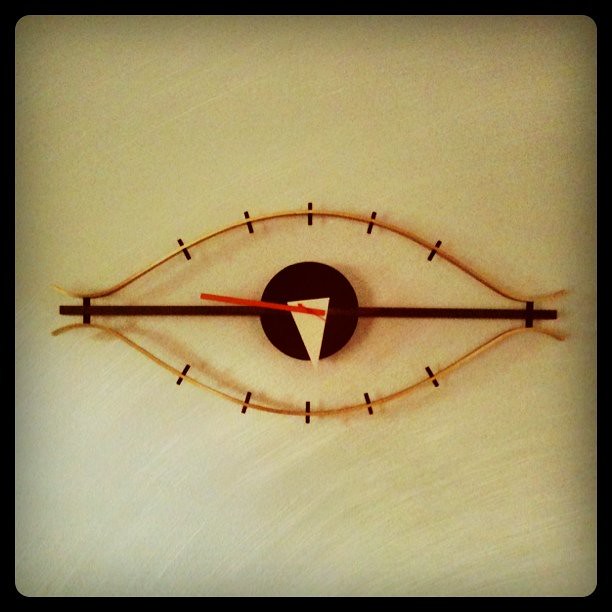This square image is framed with a narrow black border. The background presents an off-white to yellowish hue with visible brush marks, adding texture as they stretch diagonally from the upper right to the lower left, suggesting a painted wall. 

Central to the image is a uniquely designed clock. The clock features a horizontal black bar intersecting a large black circle in the middle. At the top of this circle, there is a narrow white triangle pointing downwards, indicating the clock's twelve o'clock position, with one of the clock's hands being a thin red needle.

Above this central horizontal bar, a brown arching piece extends from the left, ascending in the center before curving back down to meet the bar. Below the central bar, an identical brown piece mirrors this arch, curving downward in the center and then rising back to meet the bar. These two brown arcs collectively give the impression of an eye, with the black circle serving as the pupil.

Atop and beneath these brown arcs are five vertical, shorter bars, distributed evenly along the arches, representing the hours. This detailed design element enhances the artistic and functional appeal of the clock, making it appear both practical and visually captivating within the context of the textured background.